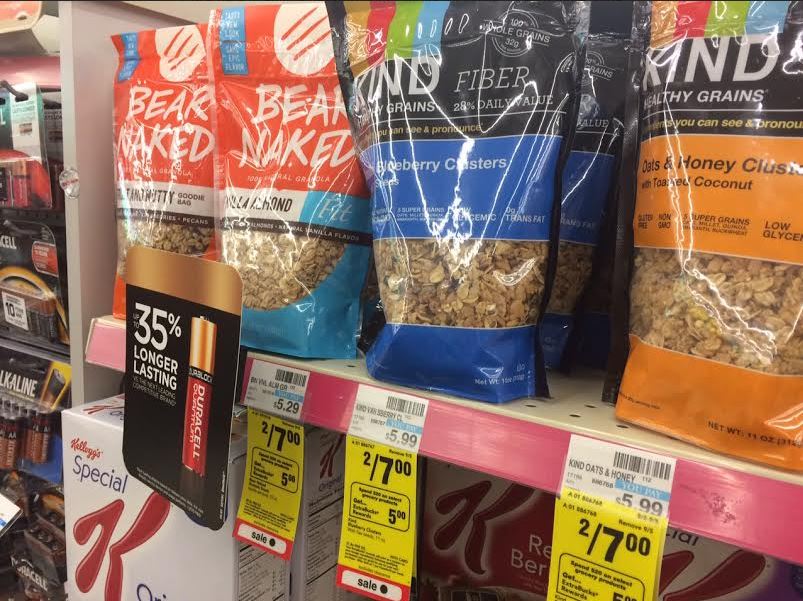The image portrays a retail shelf, likely from a CVS pharmacy based on the distinct yellow sale tags. The shelves prominently feature a selection of granola products, including "Bare Naked" and "Kind" brands. The layout includes "Bare Naked Granola" varieties in medium red and medium blue bags, showcasing flavors such as Vanilla Almond and another difficult-to-read variant due to glare. Additionally, "Kind" granola types like Oats and Honey Clusters and Blueberry Clusters are displayed in black and orange packaging. Clearly visible through the packaging are granola clusters, revealing the product within. Sale tags beneath the items indicate a price of two for $7.

Adjacent to the granola products, there is a large Duracell advertisement, emphasizing a 35% longer-lasting battery feature. To the left of the granola are partly visible battery packs. Below the granola shelf, there are boxes of Kellogg's Special K cereal, including the Original variety and potentially other types, visible in white packaging. This detailed arrangement showcases the diverse selection of snack and breakfast products available in the store aisle.